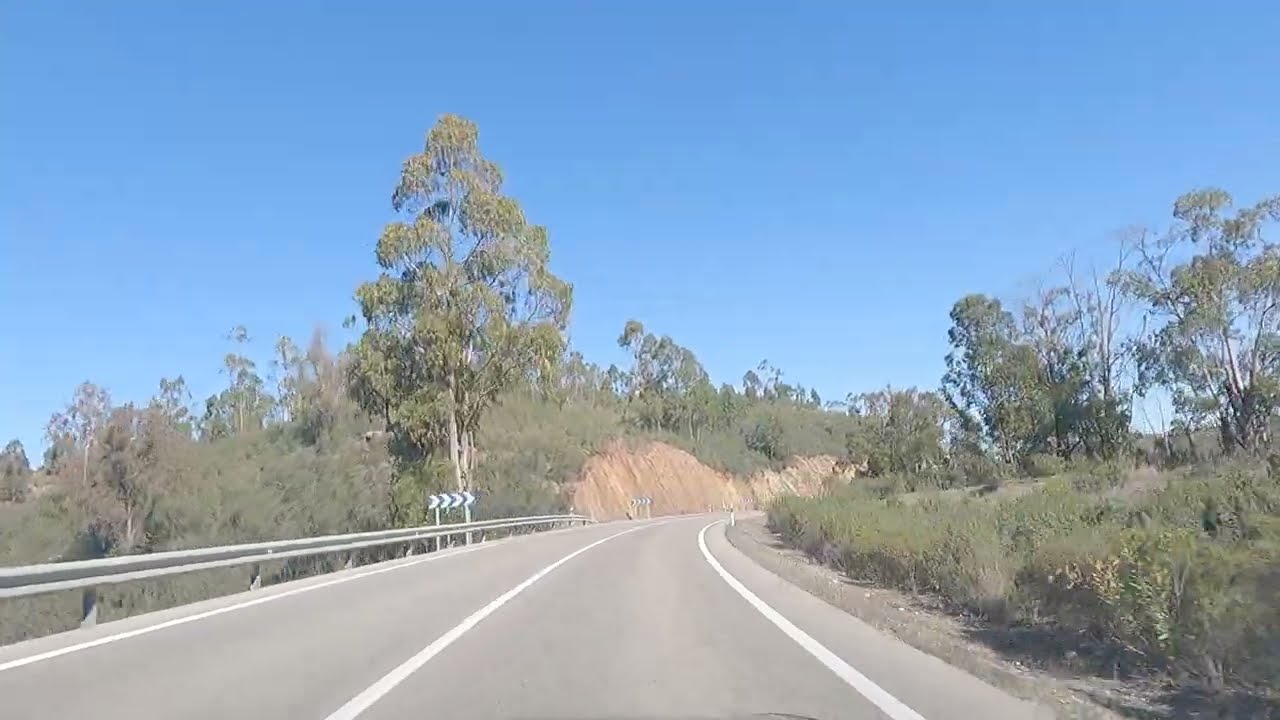This photograph captures an isolated, two-lane highway that extends from the bottom of the frame toward the center, where it curves to the right and exits the shot. The road features white paint markings indicating its sides and middle. A metal guardrail lines the left side of the road, adorned with black and white arrow signs warning of the impending right turn. Adjacent to the road are dirt and gravel shoulders, which give way to bushy green grasses and leafy trees. As the road curves, there are sandy cliffs or raised dirt on the left side, suggesting the elevation was cut through a hill. The scene is bathed in clear, sunny light under a light blue sky devoid of clouds, adding to the impression of a warm climate.